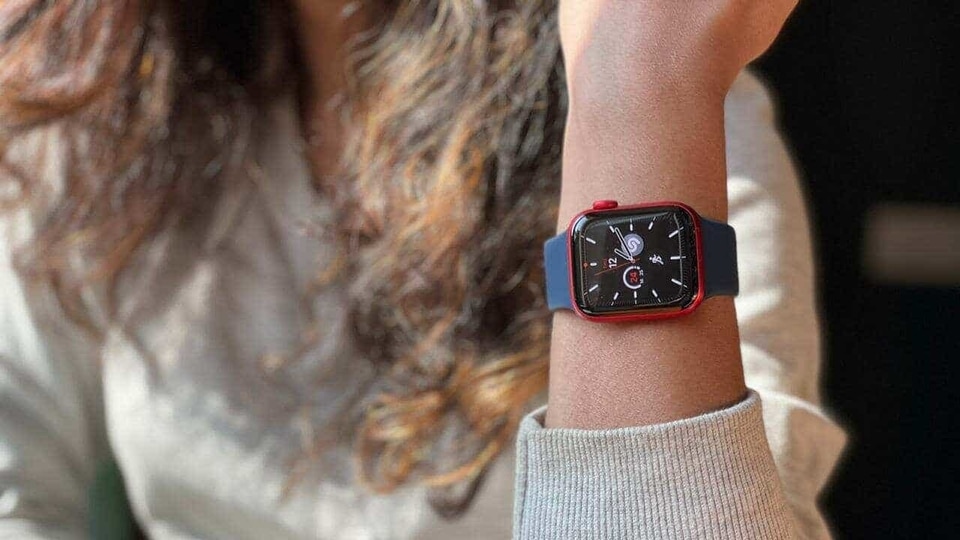The photograph captures a woman with long, wavy hair that's a mix of black and blonde, cascading over her shoulders and down to her mid-chest. She is wearing a long-sleeved white blouse and stands slightly out of focus in the background. The primary focus of the image is her left arm, which is raised upright, displaying a watch close-up. The watch, strapped to her wrist with a blue, cloth-like band, features a rectangular face with a red border around a black center. The watch face shows analog hands, with the small hand pointing at 1 and the large hand near 2. The face also includes white and black hands, line markers for the numbers, and a distinctive small red dot near where 9 would be. Additionally, there is a little red button on the top right side of the watch. Her forearm is lifted in such a way that her knuckles face upward and her elbow points toward the floor, allowing a clear view of the watch.